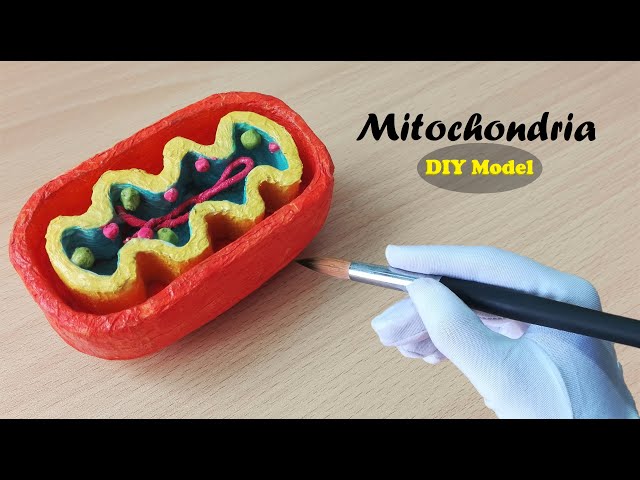The image showcases a meticulously crafted DIY Mitochondria model, likely made from either clay or styrofoam, and positioned on a wooden table. A person, wearing a blue glove, is seen holding a black-handled paintbrush, delicately painting the outer layer of the model rich red. The model takes on a pill-shaped form, with an exterior resembling an orange bowl. Inside, a yellow and intricately squiggled secondary structure is visible, which transitions to a blue interior. Embedded within the blue section are several small balls, painted green and pink, and intertwined with a similarly pink, twisted strand. This detailed project encapsulates the inner workings of a mitochondrion in a vivid and tactile three-dimensional form. The scene is likely part of an educational video or promotional content for a Mitochondria DIY model from a company named Mito Chandria, highlighted by yellow and black lettering in the background.